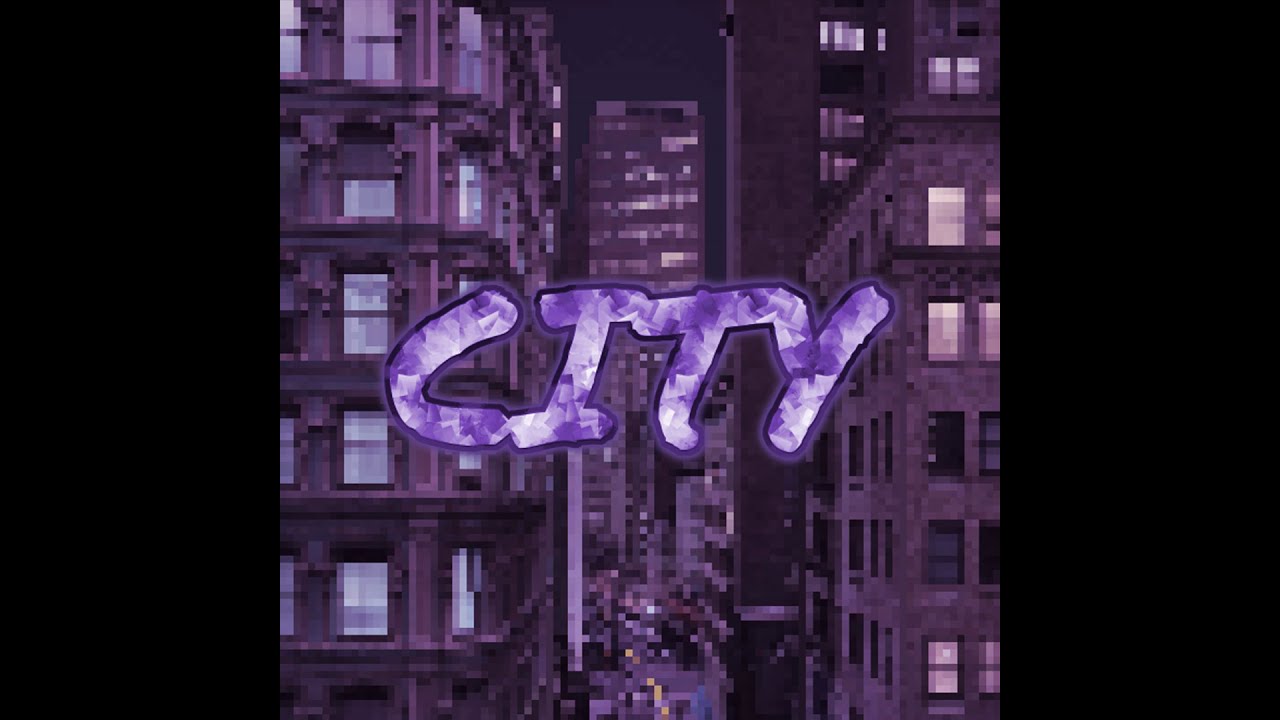The image exhibits a pixelated cityscape scene viewed between tall skyscrapers, primarily set under a darker, purplish filter that suggests nighttime. The pixelation lends a grainy, digitized appearance, giving the city a somewhat blurry and abstract look. Notable architectural details include at least three noticeable buildings: one to the left, one centrally placed, and another to the right, along with indistinct vehicles on the streets below. Dominating the center of the image, chunky, bubbly letters spell out "CITY" in capital letters. Each letter is adorned with what resembles sparkling or crystallized textures, outlined in dark purple, adding to the artistic feel of the composition. The sides of the frame are plain black, further emphasizing the central pixelated city scene. The overall effect is an intriguing blend of digital art and a stylized urban nightscape.